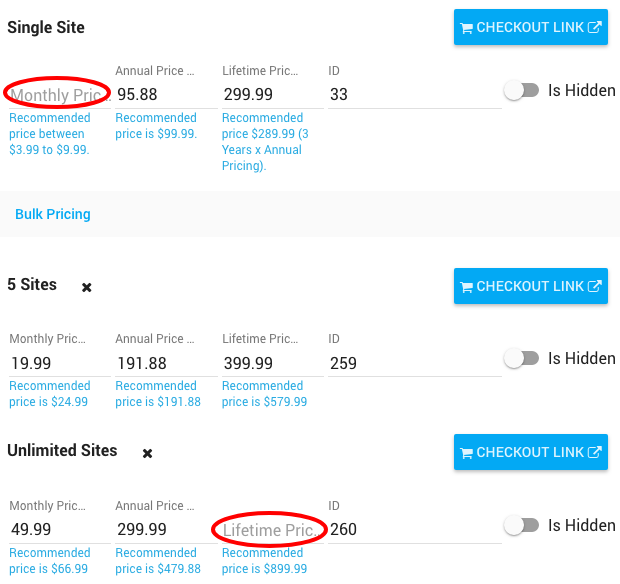**Screenshot Description: Subscription Pricing Comparison on E-Commerce Platform**

The screenshot appears to be from an e-commerce platform showcasing different subscription pricing options. Key areas are highlighted with red circles, presumably for emphasis or clarification.

**Single Site Plan:**
- **Label:** "Single Site" in black text.
- **Checkout Button:** Blue with white text and a shopping cart icon, labeled "Checkout Link."
- **Pricing:**
  - Monthly Price (cut-off, in gray text, circled in red).
  - Annual Price: $95.88.
  - Lifetime Price: $299.99.
  - ID: 33.
  - **Toggle for "Is Hidden":** Set to off.
- **Recommended Prices:**
  - Monthly: $3.99 to $9.99.
  - Annual: $99.99.
  - Lifetime: $289.99 (calculated over multiple years of annual pricing).

**Bulk Pricing Plan:**
- **Label:** "Bulk Pricing" in blue text.
- **Plan Details:** Includes coverage for five sites, indicated by a blue label with an "x5."
- **Checkout Button:** Blue with white text and a shopping cart icon, labeled "Checkout Link."
- **Pricing:**
  - Monthly Price: $19.99 (recommended: $24.99).
  - Annual Price: $191.88 (recommended: $191.88).
  - Lifetime Price: $299.99 (recommended: $579.99).
  - ID: 259.
  - **Toggle for "Is Hidden":** Set to off.

**Unlimited Sites Plan:**
- **Checkout Button:** Blue with white text and a shopping cart icon, labeled "Checkout Link."
- **Pricing:**
  - Monthly Price: $49.99 (recommended: $66.99).
  - Annual Price: $299.99 (recommended: $479.88).
  - Lifetime Price: $899.99 (circled in red) (recommended: $899.99).
  - ID: 260.
  - **Toggle for "Is Hidden":** Set to off.

This detailed screenshot provides a clear comparison of different subscription options and their respective pricing, highlighting any inconsistencies or promotions.